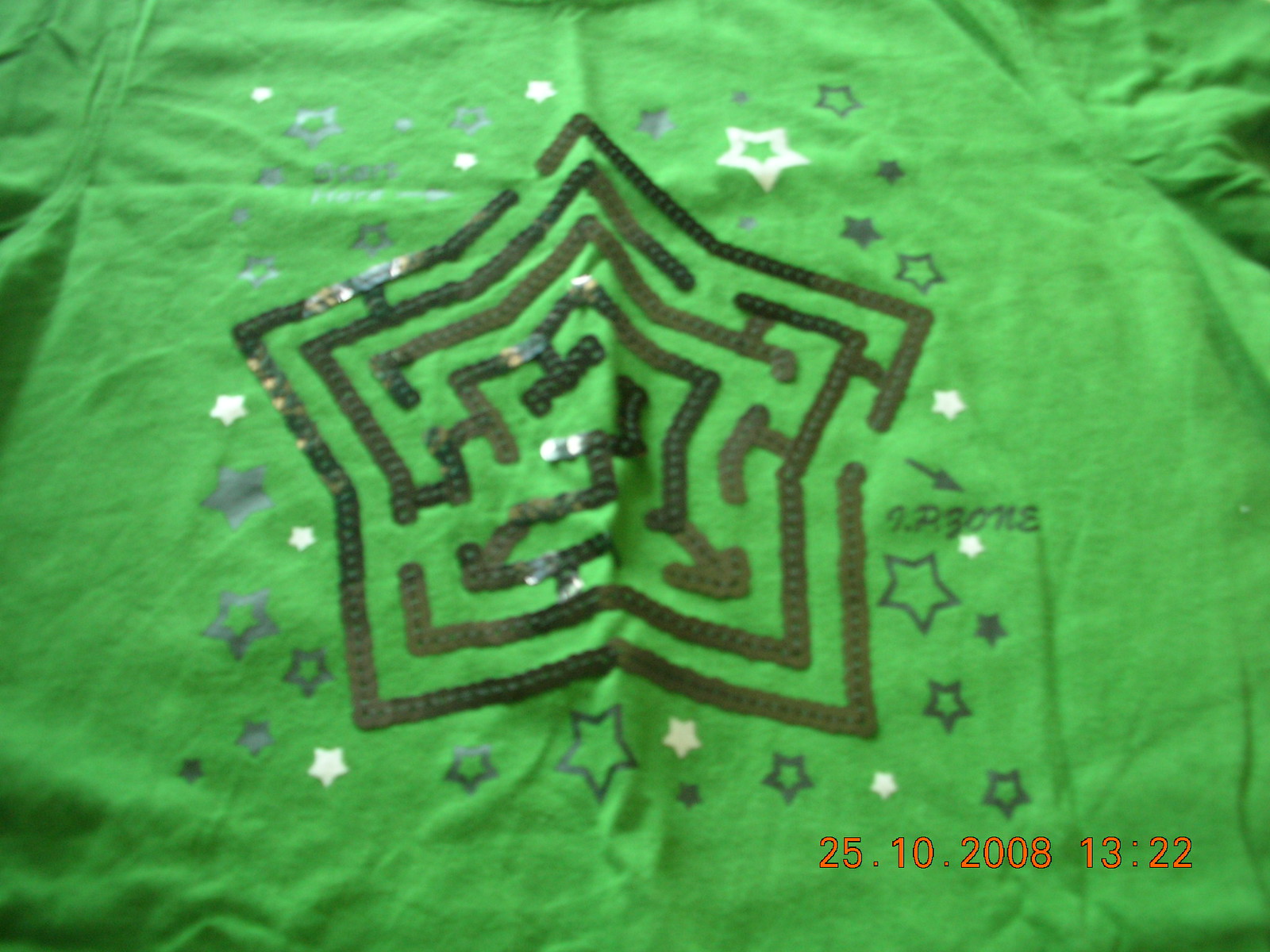This photograph captures a vibrant, child-sized shirt set against a plain background. The bright green fabric of the shirt immediately stands out due to its lively hue, though it is somewhat wrinkled. In the corners of the image, specifically the bottom right, a timestamp is visible in red text, reading "25.10.2008" and "13:22."

The shirt features a prominent, intricate design centered on its front. A large maze is displayed within a thickly outlined star, composed of a network of black lines. This maze invites one to trace their way through its labyrinthine paths. Surrounding the central star, a scattering of smaller, colorful stars in various shades of white and blue adds a playful and whimsical touch to the garment. Each smaller star varies in style, contributing to the overall cheerful and dynamic look of this bright green, eye-catching shirt.